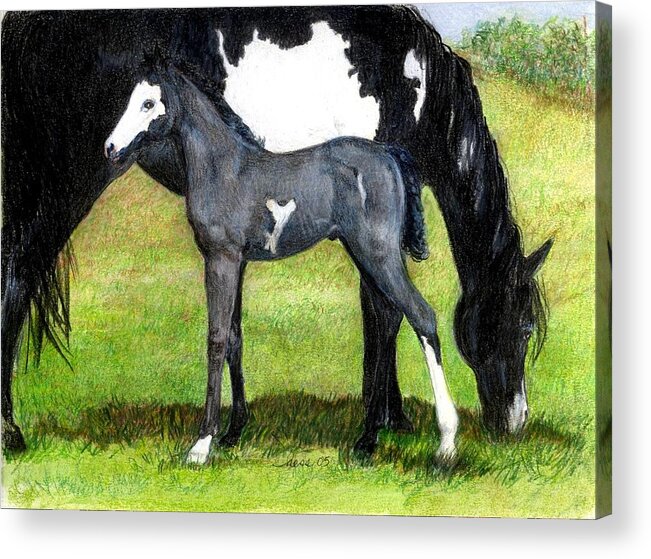This artwork is a highly detailed painting of two horses against a serene backdrop of lush green grass and a vivid blue sky. The composition showcases a smaller, black and white foal positioned centrally, distinguished by its primarily black coat, a white face around its nose and eyes, and white markings on its legs and underbelly. The foal is marked with a branding emblem in the middle of its abdomen. Beside it stands a larger horse, possibly the mother, with a mostly black coat accented by white splotches on its stomach and longer fur. This larger horse is hunched down, facing away from the foal, engrossed in grazing. Both horses exhibit a high level of detail, with fine lines suggesting the use of a small paintbrush. The painting, rendered on canvas, might be a product photo, given its slight off-center placement against a white wall.